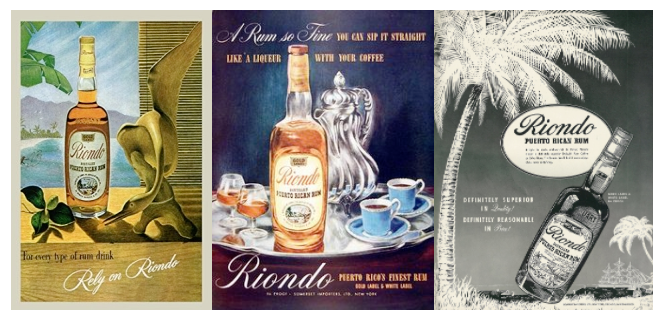The image features a detailed advertisement for Riondo Puerto Rican rum, split into three distinct parts. On the left, there's a tropical-themed poster with an orangish-yellowish background, a bottle of Riondo rum with a rose-colored liquid and a white label adorned with a circular picture. The foreground includes light wooden planks, a carved wooden bird with a long neck appearing to feed on leaves near the bottle, and scenic illustrations of a beach, ocean, palm trees, mountains, and a small person approaching the water in the distance. The middle section of the advertisement is more elegant and sophisticated, showing a silver serving tray with two blue and white teacups on the right, and two snifters filled with Riondo rum on the left. The text above reads "A rum so fine, you can sip it straight like a liqueur with your coffee," with "Riondo, Puerto Rican's finest rum" written below, highlighting both gold and white labels. The rightmost part of the ad is a black and white image featuring a palm tree, a tilted Riondo bottle, and a ship in the background. A white oval stamp declares "Riondo, Puerto Rican rum," with additional text boasting the rum's superior quality and reasonable price.